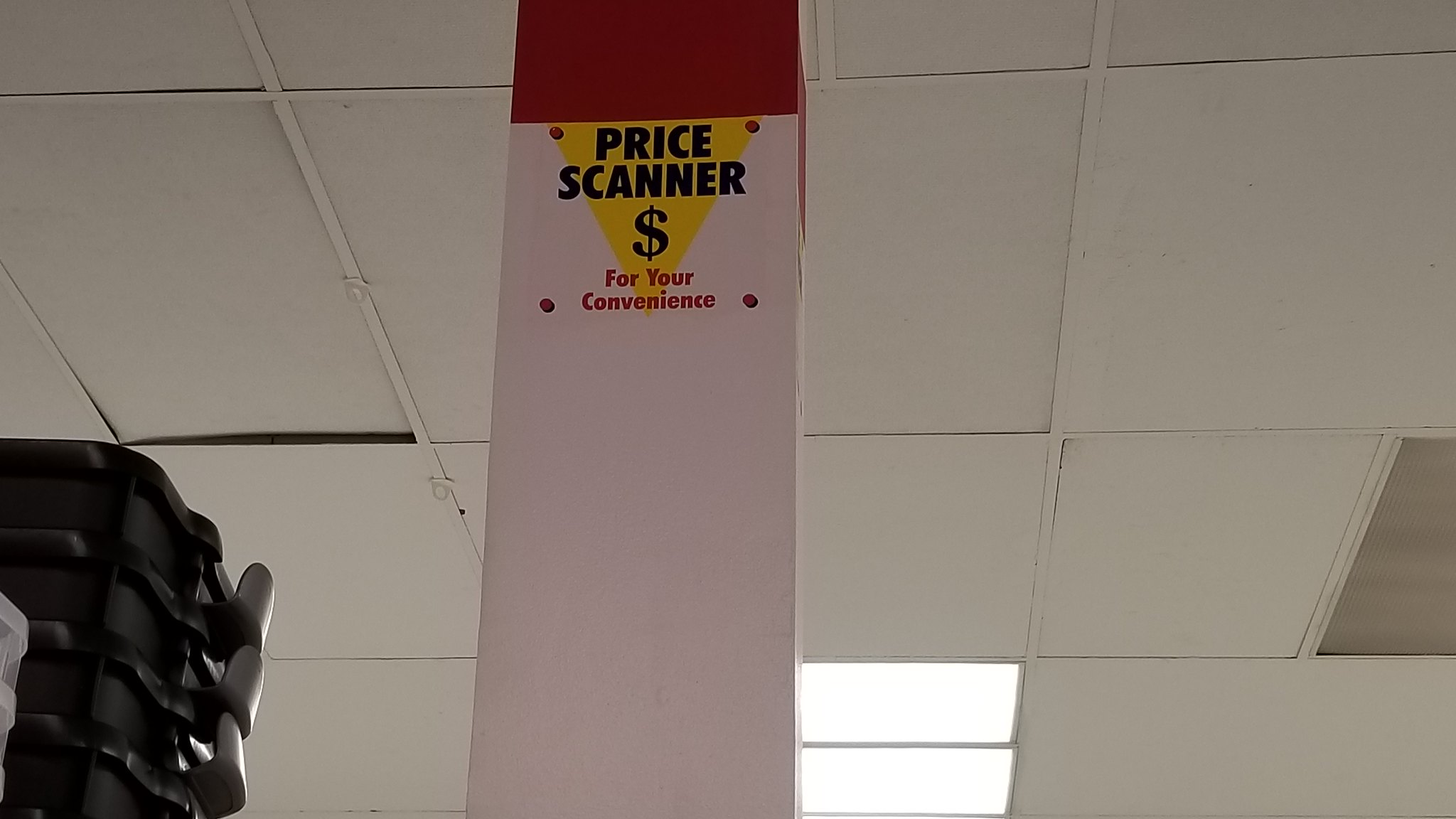The image captures an interior view of a store from an upward-looking perspective, focusing on a structural pillar that supports the roof. The ceiling surrounding the pillar is composed of white or off-white tiles set into rectangular frames made of white-painted metal. The lighting is provided by semi-translucent panels with lights behind them; only two of these panels are illuminated, emitting a white light, while a third light panel remains off. 

In the bottom left corner of the image, there are several black buckets or containers, possibly rubbish bins, stacked together, each featuring silver handles. The pillar in the center of the image is painted red and white and has a sign attached to it. The sign has a white background with black text that reads "Price Scanner," accompanied by a dollar sign in red. Behind this message is a yellow inverted triangle.